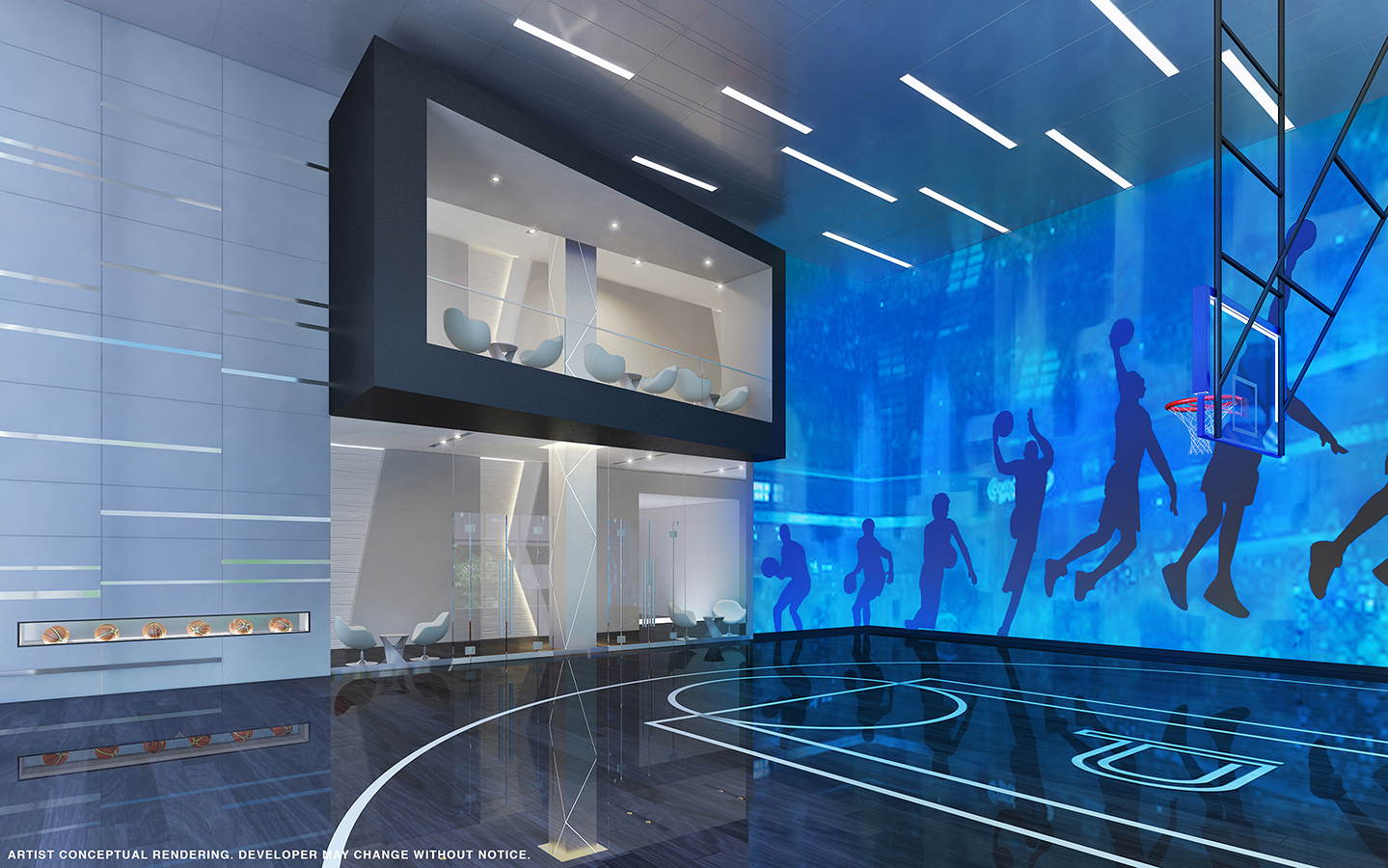The image illustrates a futuristic, sophisticated gym, showcasing a conceptual rendering of a specialized basketball practice court designed by an artist, prominently noted with the text "Artist's conceptual rendering, developer by chance without notice." The court features a half-court layout with a sleek black surface, accentuated by stark white lines marking the boundaries and a distinctive ‘P’ or ‘D’ at the center of the restricted area. The lone basketball hoop stands on the left-hand side, meticulously detailed almost as if it has been photoshopped into the scene. The ambiance is enhanced by modern, futuristic elements: the left wall boasts horizontal white and silver accents on large tiles, featuring a rectangular window displaying six basketballs, possibly mirrored. Above the court, elegant box seats with six chairs each overlook the training area, flanked by two lounge areas filled with contemporary white egg chairs.

Dominating the far wall is a striking blue mural, portraying a sequence of dark blue silhouettes of a player dribbling and executing a dunk, captured in seven progressive stages against a lighter blue backdrop. This dynamic artwork adds a sense of motion and energy to the space. Enhanced by creative and funky lighting throughout the facility, the setting merges athletic functionality with modern design, embodying a new-age creation that seems almost surreal.